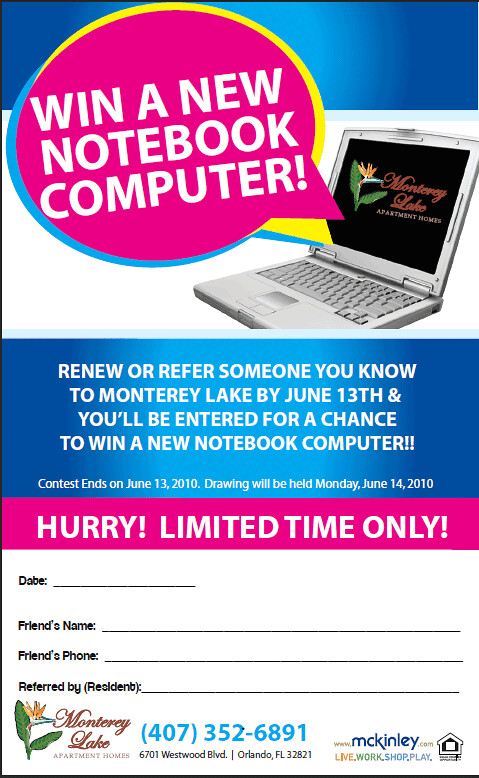This advertisement poster features a chance to win a new notebook computer. At the top, it displays an image of a silver laptop with the company logo and name "Monterey Lake" on its screen. To the left of the laptop is a circular pink word bubble with the text: "Win a New Notebook Computer." Below this, against a blue background, the advertisement reads: "Renew or refer someone you know to Monterey Lake by June 13th and you will be entered for a chance to win a new notebook computer. Contest ends June 13th, 2010. Drawing will be held Monday, June 14th, 2010." Below the blue section, a red strip contains the urgent message: "Hurry, limited time only." The lower part of the poster features a blank form for participant details against a white background, asking for the date, friend's name, friend's phone, and the person referred by. Also included are various logos and contact information such as phone numbers and the website mckinley.com.